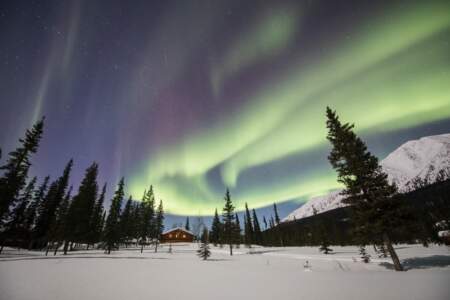This digitally-altered, horizontally-oriented photograph captures a serene, snowy landscape under the vibrant display of the northern lights. Dominating the foreground is a flat, untouched field of fresh snow, dotted sporadically with dark green pine trees, which become more numerous and taller towards the left of the image. Centered horizontally but slightly off to the left and about 50 feet into the scene, a small red wooden cabin with orange lights acts as a focal point, its rustic charm contrasting with the ethereal surroundings.

To the right of the cabin, the landscape features a darker slope leading up to a majestic, snow-covered mountain. The sky above is awash with northern lights, displaying an array of colors from light green streaks to darker purple stripes. These vibrant hues fade from a deep purplish sky with shades of turquoise green that stretch from the center towards the right, mingling with bands of pink. The surreal quality of the sky casts doubt on whether it is day or night, adding to the mystique of the scene. The overall composition, framed by the illuminated winter sky and the placid snow-covered terrain, evokes a tranquil yet captivating Arctic atmosphere.